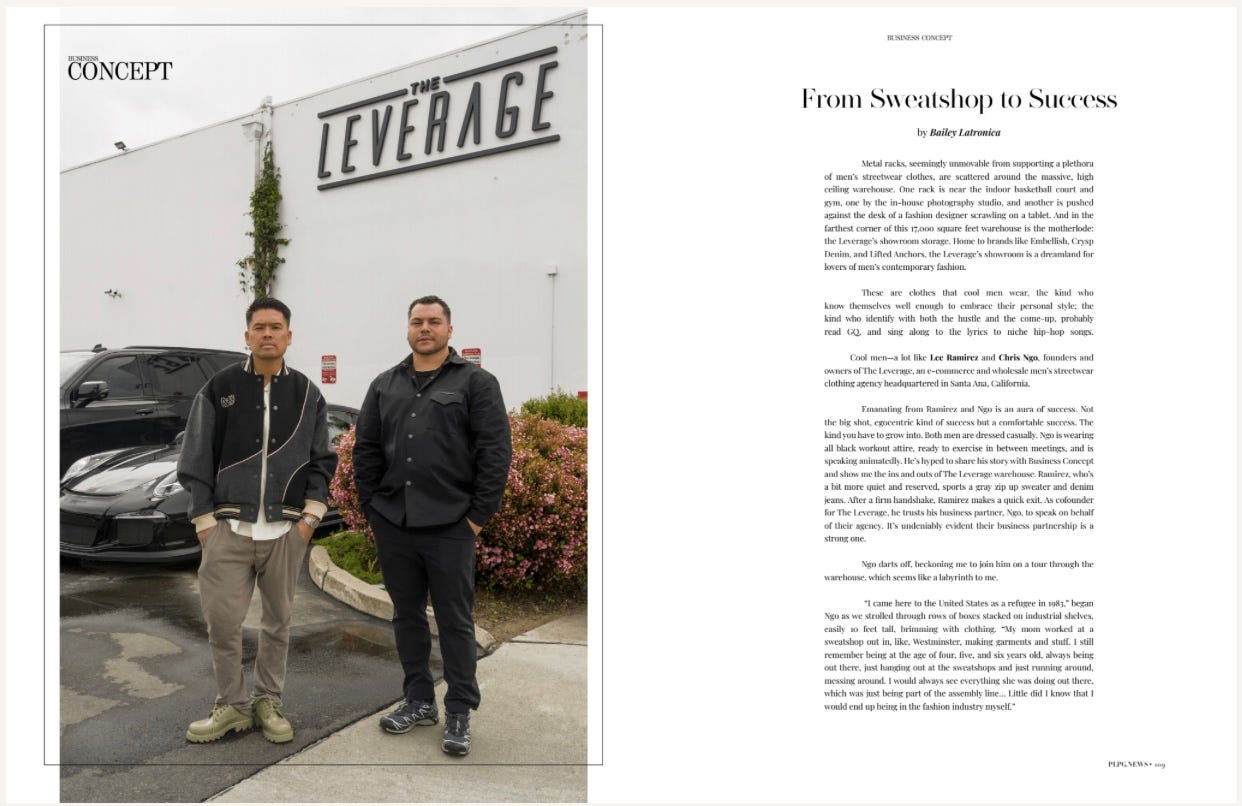The image, taken from a magazine, is divided into two parts. On the left side, a photograph captures two men standing in a parking lot in front of a building labeled "The Leverage." Both men, of average height and brown-haired, are dressed in dark clothing suitable for cooler weather, each with their hands in their pockets. The man on the left wears a gray and black zip-up jacket, tan pants, and tan boots, while the man on the right sports a black button-up shirt, black pants, and tennis shoes. Behind them, a bush with flowers, a touch of grass by the curb, and two cars – a black sports car and a black SUV – are seen. The top left corner of the photo indicates it’s part of a section called "Business Concept."

On the right side, there is an article titled "From Sweatshop to Success" by Bailey Latronica. Though the text is mostly unreadable due to its small size, some lines describe a scene inside a high-ceiling warehouse filled with metal racks of men's streetwear, an indoor basketball court, a gym, a photography studio, and a fashion designer's workspace. The background of this page is white.